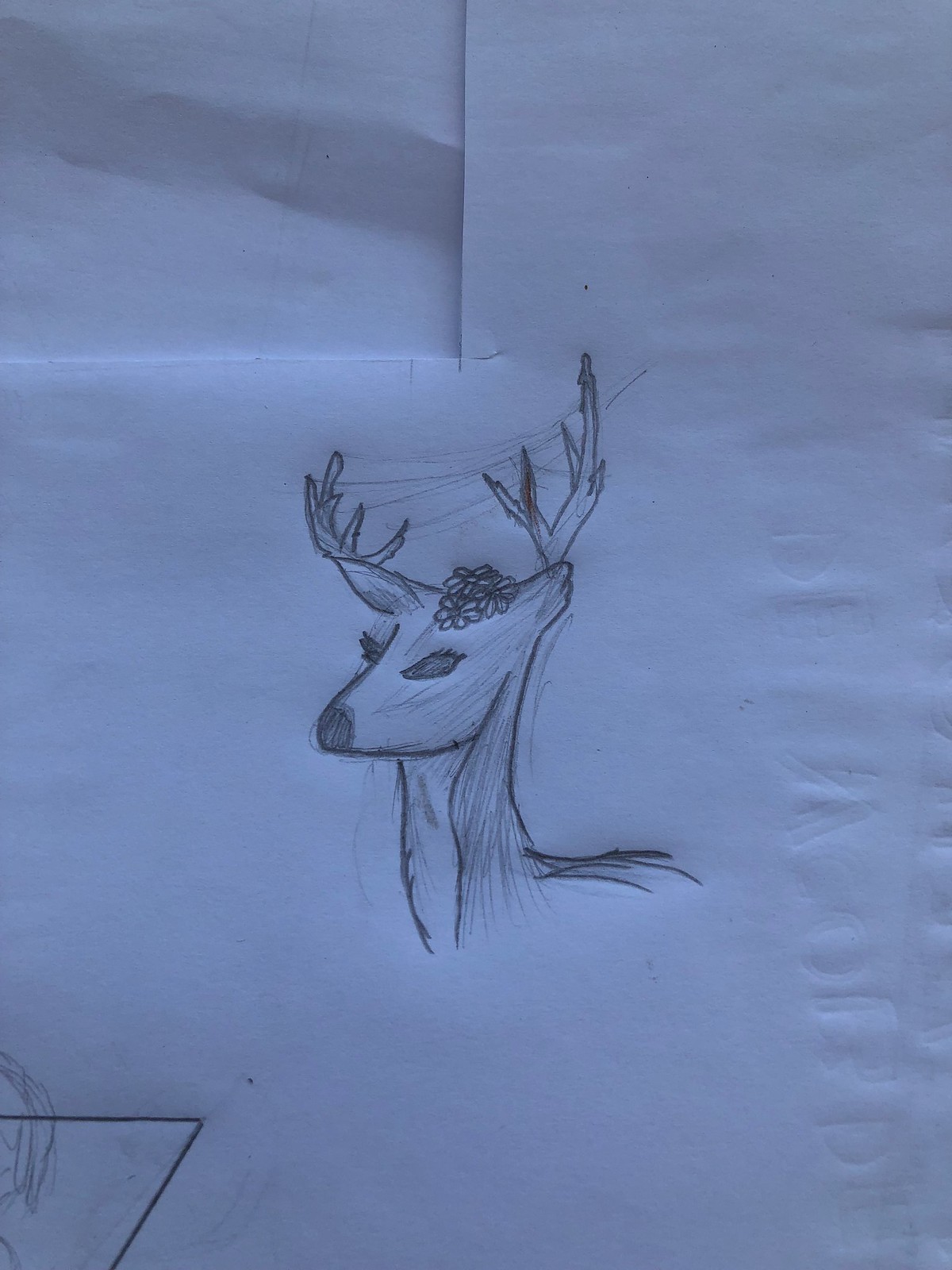This image is a lightly sketched pencil drawing featuring the head, neck, and upper torso of a buck with antlers. The drawing is centered on a piece of plain, unlined paper, appearing slightly blue-tinted as if photographed in low light without a flash. The buck is depicted with almond-shaped, slanted eyes and a clearly defined nose. There are visible textures in the fur, achieved through soft lines and shading, especially in the neck area, while the throat and chest remain plain white.

Atop the buck's head rests a decorative design of three flowers. The antlers, originating from the top of the head, are simply sketched and short. In the lower right corner of the image, there is a triangular shape with thicker lines, possibly part of an incomplete doodle. Additionally, indentations on the paper suggest it was used as a support while something was written on an overlying sheet. The top left corner of the paper appears altered, as if it had been folded and then cut.